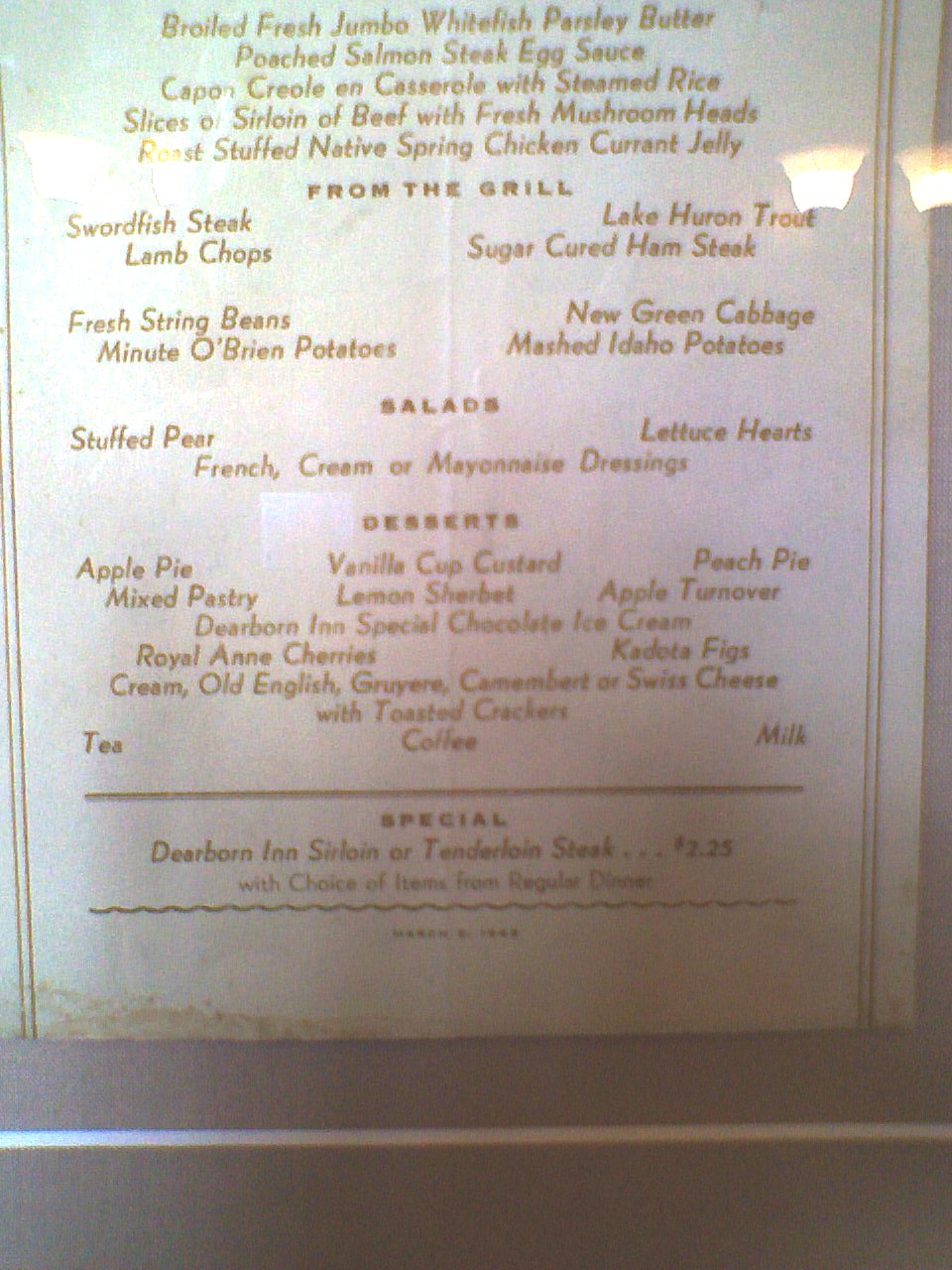This image captures an elegant menu displayed on a wall, likely within a restaurant setting, although the precise location—inside or outside—remains unclear. A subtle reflection of a sophisticated floor lamp with a warm white and yellow glow adds a touch of ambiance to the scene. The menu appears well-protected from the elements, suggesting a deliberate effort to maintain its pristine condition.

The restaurant’s name is not visible, but the offerings suggest a high-end dining experience. Detailed descriptions of menu items include:

- **Broiled Fresh Jumbo Whitefish with Parsley Butter**
- **Poached Salmon Steak with Egg Sauce**
- **Capon Creole in Casserole with Steamed Rice**
- **Slices of Sirloin of Beef with Fresh Mushroom Heads**
- **Roast Stuffed Native Spring Chicken with Currant Jelly**

These dishes seem to be part of the main course selections rather than samples or appetizers.

The menu is elegantly written in a medium brown, non-cursive font. The section "From the Grill" includes:

- **Swordfish Steak**
- **Lamb Chops**
- **Lake Huron Trout**
- **Sugar-Cured Ham Steak**

The sides are listed in two columns, featuring:

- **Fresh String Beans**
- **New Green Cabbage**
- **Fried O'Brien Potatoes**
- **Mashed Idaho Potatoes**

Under "Salads," the menu offers:

- **Stuffed Pear**
- **Lettuce Hearts with French Cream or Mayonnaise Dressings**

The "Desserts" section is creatively formatted, almost in three columns, listing:

- **Apple Pie**
- **Vanilla Cup Custard**
- **Peach Pie**
- **Mixed Pastry**
- **Lemon Sherbet**
- **Apple Turnover**
- **Dearborn Inn Special Chocolate Ice Cream**
- **Royal Anne Cherries**
- **Kadoda Figs**
- **Cream**
- **Old English, Gruyere, Camembert, or Swiss Cheese with Toasted Crackers**

Tea, coffee, and milk are also available.

Interestingly, no prices accompany the menu items, except for a special dish at the very bottom: the "Dearborn Inn Sirloin or Tenderloin Steak with a Choice of Items from the Regular Dinner" priced at $2.25. This pricing suggests the menu is from a bygone era, where such a luxurious meal would now likely command much higher prices.

The menu's intricate detailing and high-quality offerings indicate a refined dining experience, possibly at a historical establishment like the Dearborn Inn.